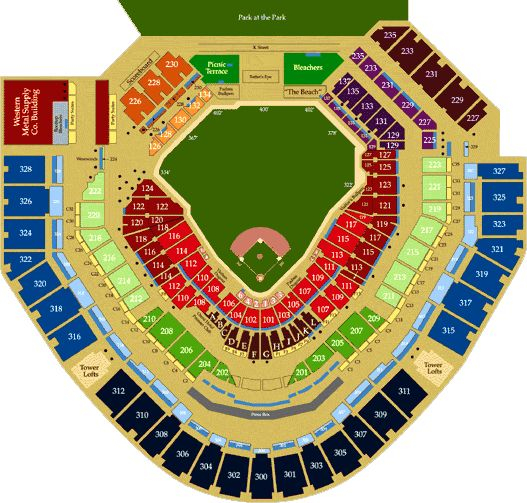The image depicts a vivid and detailed graphical illustration of the seating arrangements in a baseball stadium. Central to the image is the iconic diamond-shaped green field, epitomizing the heart of the ballpark. At the top of the illustration, a green banner with the phrase "Pack at the Park" boldly written in white, frames the scene.

Surrounding the baseball field, diverse layers of rectangular shapes represent the various seating sections. Closest to the field is an inner layer painted a vibrant red, encircled by another layer of a reddish-brown hue. Beyond this, there are two concentric layers in different shades of green, followed by an outermost layer showcasing a gradient from lighter blue to darker blue. Each colored rectangle corresponds to distinct seating areas and is labeled with white numbers to denote specific sections.

The meticulous arrangement and color-coding of these sections provide a clear and organized representation of the seating layout, enhancing the viewer's understanding of the stadium's design.